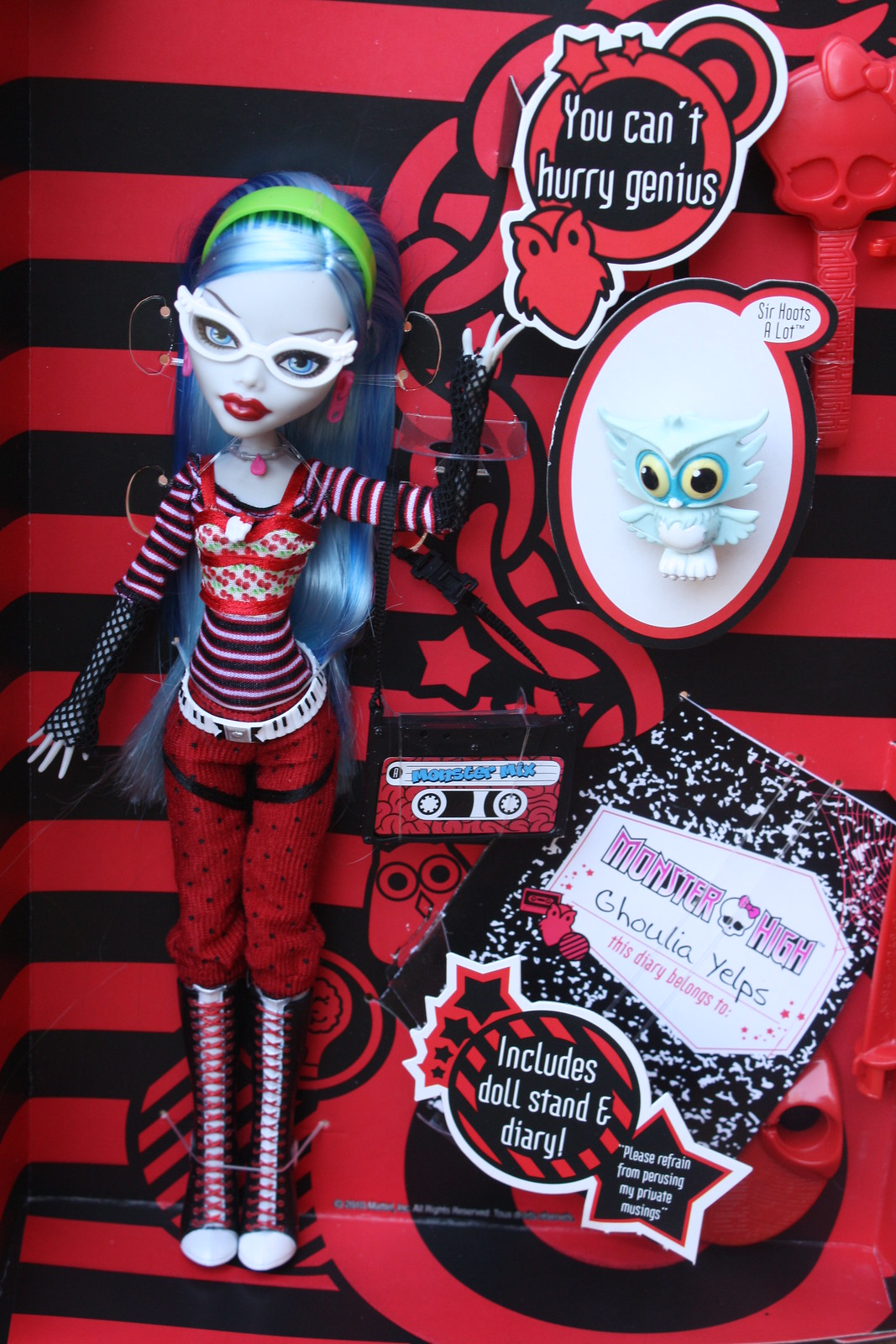The image features a promotional ad for a collectible Monster High doll, designed for edgy, pre-teens and teens frequenting stores like Hot Topic. The ad has a visually busy and jumbled layout with a striking red and black horizontally striped background.

The focal point of the image is the doll, positioned on the left side. She has long silvery purple hair and wears beige horn-rimmed glasses that obscure her ethnicity. Her attire is devilish and emo-inspired: a three-quarter sleeve sweater with red, white, and black horizontal stripes, fishnet gauntlets from elbows to wrists, and red knee-length knickers. She completes her look with red and white striped socks and white shoes.

Surrounding the doll on the right are various thematic accessories and graphics. At the top, a blurb reads, "You Can't Hurry Genius," accompanied by a red and black rendering of an owl. Below this, a white oval outlined in red and black houses a small owl figurine. Adjacent to this oval is a cassette tape with a red and black label, and further down, a gray and white marbled composition book. Superimposed on this book is a circular logo with stars, containing bold white text that reads, "Includes Doll Stand and Diary," over a red and black diagonally striped background. To the right of this circle is a large star with an illegible black and white text due to its small size.